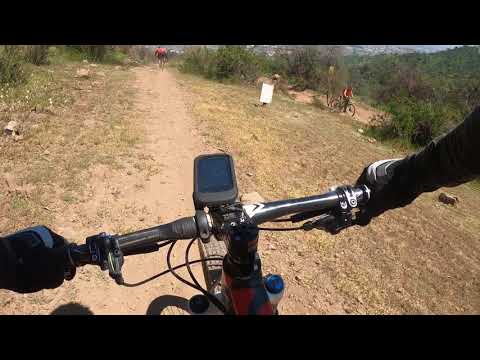The photo captures a vibrant scene from a cyclist's point of view, with the immediate focus on the black handlebars adorned with a biking computer at the center. The cyclist’s hands, clad in black gloves with a distinct silver strip, grip the handlebars firmly. The narrow dirt trail stretches ahead, flanked by patches of green bushes and leading through sunlit terrain with scattered rocks and foliage. In the forefront, the shadow of the front wheel is visible on the ground. Ahead on the path, another cyclist in a red shirt is clearly seen, while further in the distance along a rightward curve at a lower elevation, there's another rider, also donned in red. To the right side of the trail, a small white sign can be spotted amidst the grassy area. The scene is bright, with the sunlight casting minimal shadows, illuminating the entire landscape rich with trees and open sky.